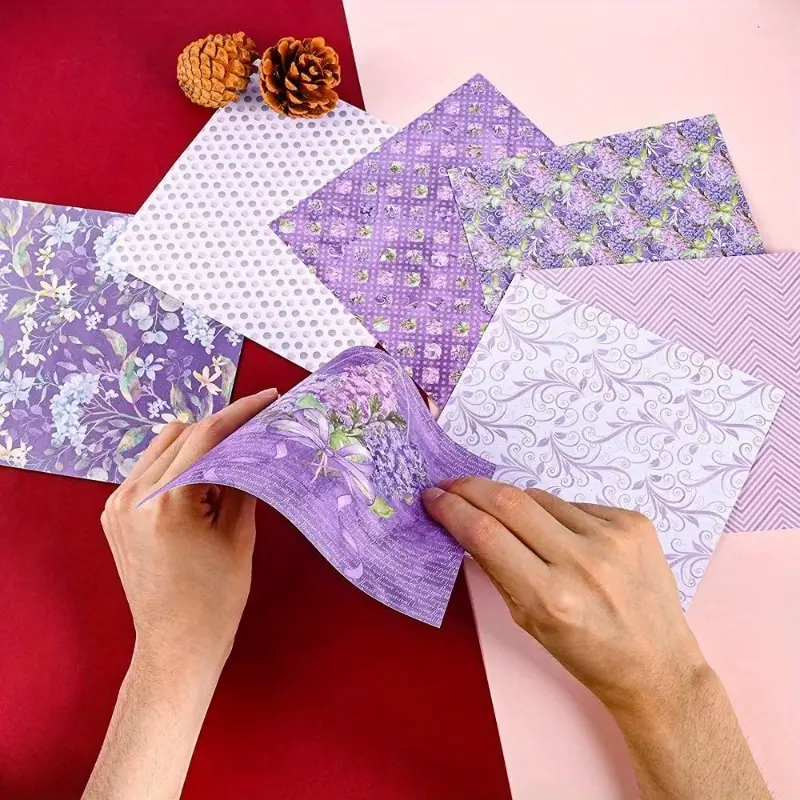This is a large square picture featuring two slender, masculine hands working with a piece of craft paper on a table. The background surface is half dark red and half pink. The person is holding a purple rectangular piece of paper adorned with a ribbon and lilac flowers, partially bent in his hands. Scattered on the table are seven different pieces of paper, each with unique designs that are mostly floral. These include a purple paper with lilac flowers and green leaves, a white paper with silver and gray polka dots, a purple paper with various flowers and square patterns, another purple paper with flowers and green leaves, a paper with purple and white zigzag lines, and a purple pattern on a white background. Adding a touch of nature to the composition, two brown pine cones sit in the upper left side of the image against the dark red background.